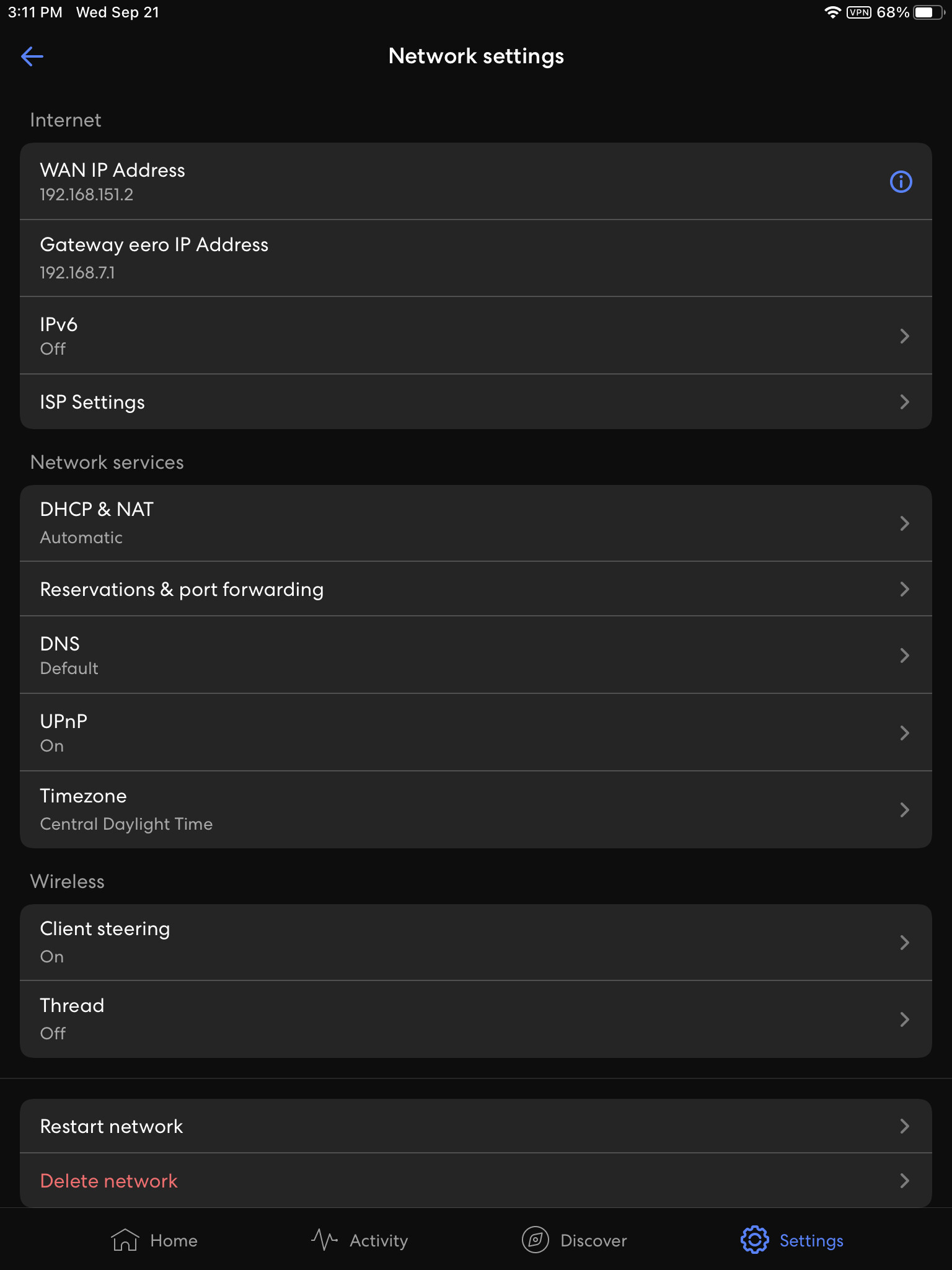A screenshot of a phone's screen displaying the network settings. At the top, the status bar shows the time (3:11 p.m.), the date (Wednesday, September 21st), and various indicators including VPN usage and a battery level at 68%. Below the status bar, "Network Settings" is centered and displayed in white text. The primary section displayed pertains to internet details, showing the IP address, Eero IP address, with IPv6 turned off and ISP settings available for further details. 

Following this, the "Network Services" section lists the current configurations: DHCP and NAT are set to automatic, Reservations and Port Forwarding are accessible, DNS is set to default, UPnP is enabled, and the time zone is Central Daylight Time. The wireless settings indicate that client steering is enabled while the thread feature is disabled. Options to restart or delete the network are also available.

At the bottom of the screen, a navigation bar features four icons: Home, Activity, Discover, and Settings, with the "Settings" icon highlighted in blue, indicating the current view. Various settings can be further explored or modified by tapping on the accompanying arrows.